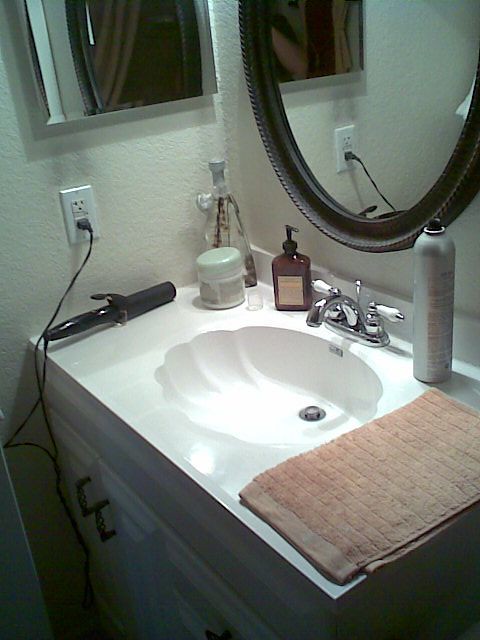In a well-organized restroom, a pristine white porcelain sink sits as the central feature. The sleek counter seamlessly transitions into the basin, where a shiny silver faucet is prominently positioned, ready to dispense water. The faucet includes two elegant handles, adorned with ivory details, to control the hot and cold water.

On the right side of the counter, a neatly folded brown towel rests beside a tall can of hairspray, suggesting a grooming routine. The left side of the sink hosts a black curling iron, plugged into the wall, likely prepped for use. At the back of the sink, a brown bottle with a black pump stands, possibly containing soap, lotion, or another beauty product.

Hovering above the sink is a round mirror with an elegant oval wooden frame. In the background, to the left of this main mirror, the lower portion of a mirrored medicine cabinet can be seen, adding functionality to the aesthetic space.